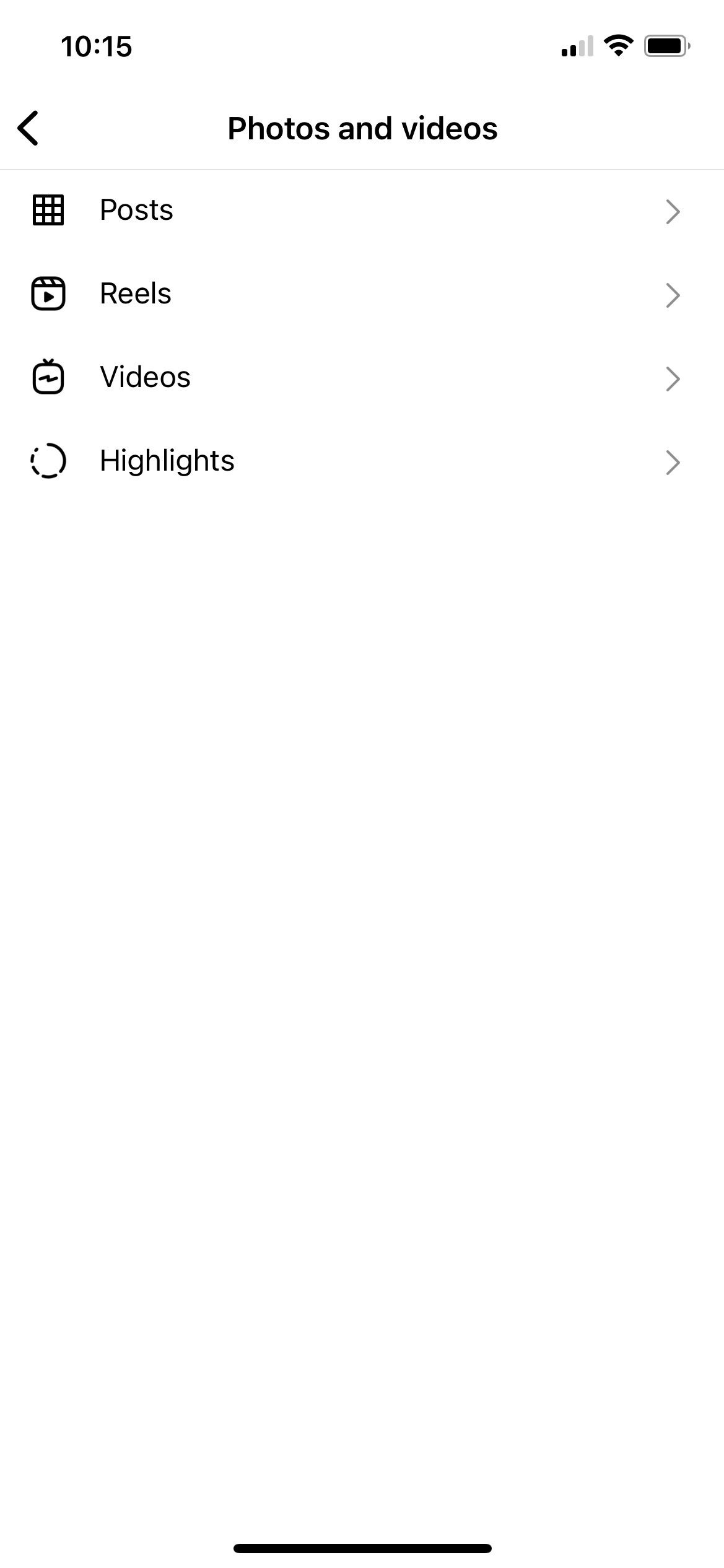The image is a screenshot taken from a smartphone. In the top left corner, the time is displayed as 10:15. Adjacent to this, the phone's signal strength shows a couple of bars, though the device is connected to a Wi-Fi network, which has full bars. The battery level is nearly full as well.

Beneath this status bar, the interface appears to display a section titled "Photos and Videos." There's a back arrow allowing for navigation to a previous screen. 

Under the main heading, there are several sub-categories listed, each accompanied by a small arrow indicating expandable options:
1. **Posts**: Marked by an illustrative graph.
2. **Reels**: Similarly expandable with an arrow.
3. **Videos**: Includes an arrow for further navigation.
4. **Highlights**: Indicated with a circular icon and an arrow for more options.

The layout and structure appear quite standard and familiar across many social media platforms, suggesting a user-friendly approach typical of apps like Facebook, although there's no definitive branding to confirm this.